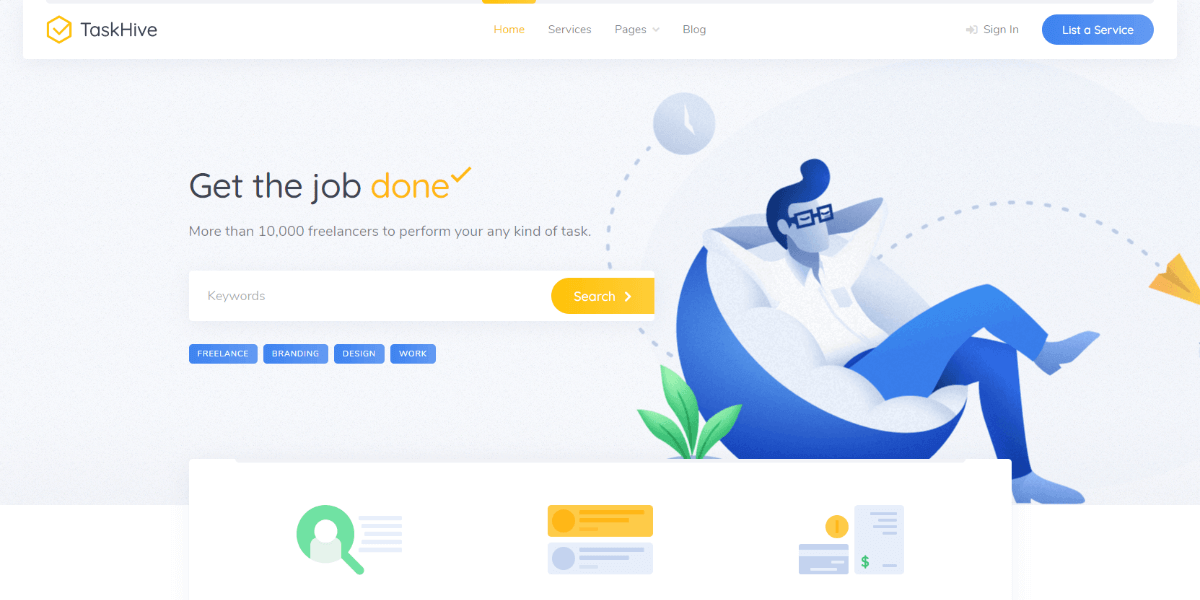The image showcases the homepage of the Tazkive website. The website features a sleek design with a dominant color scheme of white and blue, accented by yellow highlights. On the top-left corner, there is the Tazkive logo, followed by a distinct yellow hexagon symbol with a check mark inside it. 

Adjacent to the logo are navigation tabs labeled Home, Services, Pages, and Blog. The current active tab is Home, highlighted in yellow. To the right of these tabs is a sign-in option, along with a blue, oblong button labeled "List of Service."

Centrally, the homepage prominently displays a minimalist illustration of a man with a pompadour hairstyle, depicted without a mouth, sitting in a blue and white chair. Yellow arrows and a paper plane motif emanate from around him, adding a dynamic element to the composition. Overlaying this graphic is the bold headline "Get the Job Done," with the word "Done" and its accompanying check mark rendered in yellow.

Below the main headline, a byline reads, "More than 10,000 freelancers to perform any task." Further down, there is a text box for keyword searches labeled "Search." Beneath this search box, four additional navigation tabs are listed: Freelance, Branding, Design, and Work. Completing the visual setup, there is a box at the bottom containing a variety of icons, which likely represent different service categories or features.